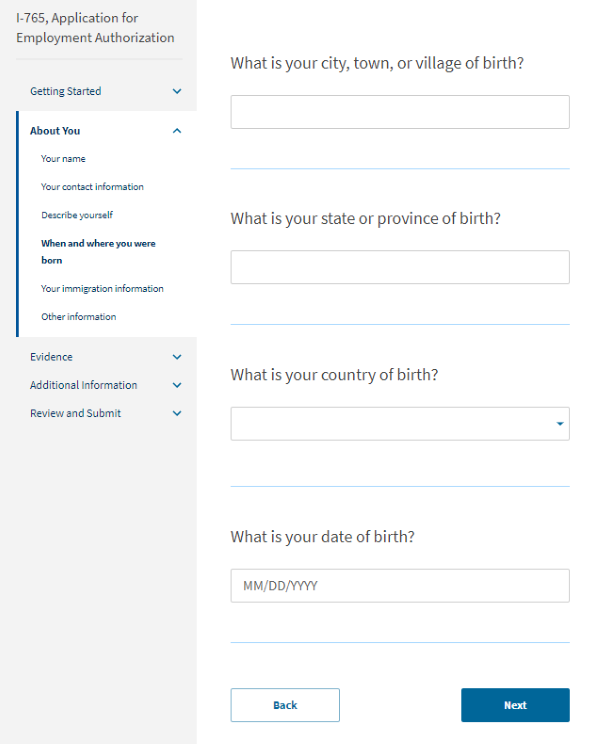This image features a digital version of the I-765 Application for Employment Authorization form. The background is primarily white, accented with shades of gray and blue, providing a clean and organized interface. 

On the left-hand side, a navigation panel aids users in progressing through the form. The sections in this panel include "Getting Started," "About You," "Evidence," "Additional Information," and "Review and Submit." Under the "About You" section, users can find subsections for entering their name, contact information, descriptive information about themselves, birth details, immigration information, and other pertinent personal information.

The main content area occupies the right-hand side of the screen, featuring a series of questions with corresponding text boxes for users to input their answers. The questions listed are:
1. What is your city, town, or village of birth?
2. What is your state or province of birth?
3. What is your country of birth?
4. What is your date of birth?

The interface is designed to gather essential personal information typically required for employment authorization applications, following a structured and user-friendly format for easy completion.